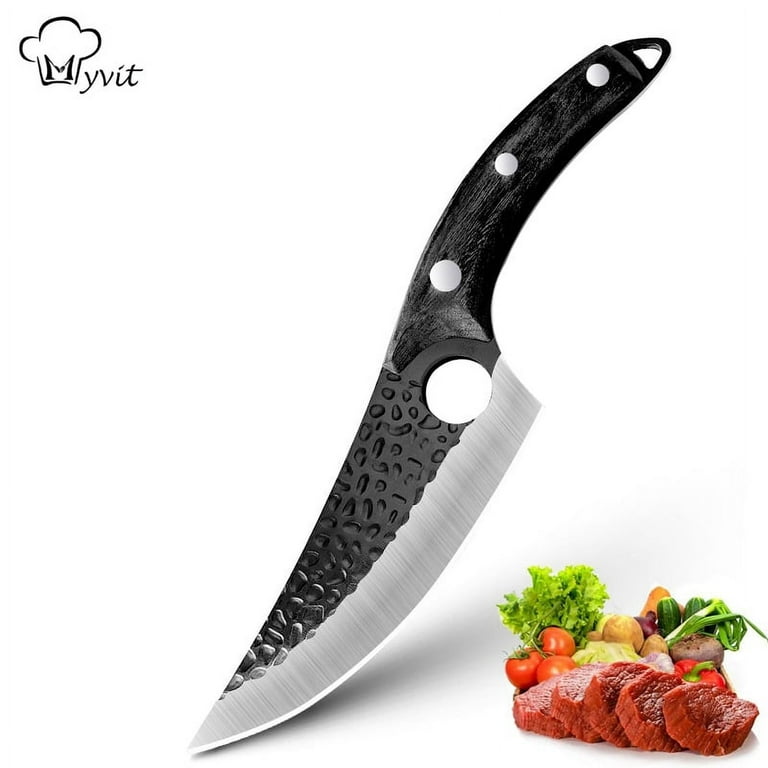This detailed image showcases a sleek and stylish kitchen knife prominently set against a blank white background. The upper left corner features the brand icon, which includes a stylized letter 'M' inside an outline resembling a broccoli crown, part of a logo that reads "MyVIT". This logo suggests a culinary theme.

At the center of the image is the knife, which boasts a modern and ergonomic design. The blade is distinctly two-toned: the top half is black with artistic indentations, while the bottom half is a polished silver. The shape of the knife is unique, with a curved blade that sweeps slightly downward and then sharply back up towards the tip. The handle, mimicking the blade's S-curve, appears to be made of a synthetic material with an artificial wood grain texture, and it is secured with polished silver bolts. A noteworthy feature of the knife is the circular hole located at the back of the blade, near the handle, which adds to its aesthetic and functional design.

To the right of the knife, there is an assortment of fresh produce intended to highlight the knife's cutting capability. This includes greens, potatoes, green onions, mushrooms, tomatoes, and potentially some cabbage. In the foreground, five slices of red meat are displayed, emphasizing the knife's sharpness and precision.

Overall, this image effectively combines the elements of branding, product design, and practical use, illustrating both the elegance and functionality of the MyVIT kitchen knife.